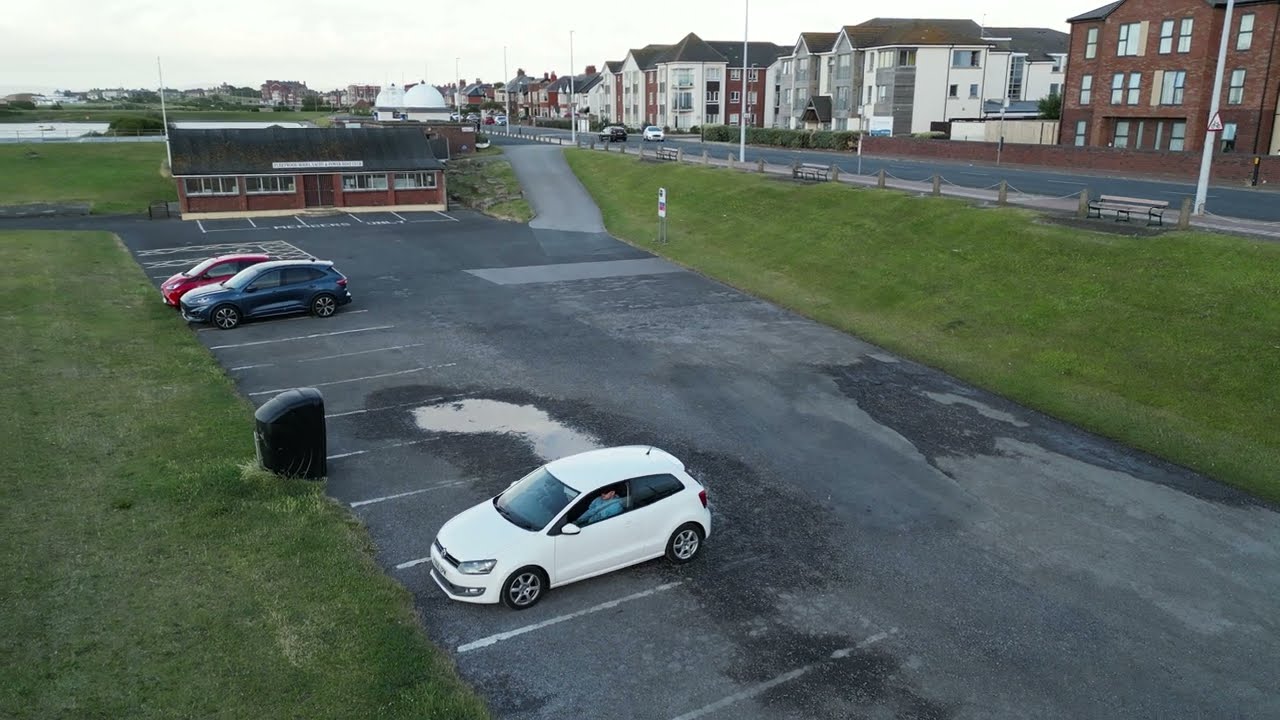The image captures an outdoor parking lot from an elevated perspective, possibly from a drone. The main focus is a white hatchback car with its windows halfway down and an individual sitting in the driver’s seat. Adjacent to the white car, there are two other vehicles: a blue four-door vehicle and a smaller red two-door vehicle. A black garbage can is situated off to the side, near the middle row of parking spaces.

To the left of the parking lot stands a small brown building with several windows, potentially an office building, though its exact purpose is unclear. A small access road beside the building leads up a grassy hill with a partially visible sign, and further up, the road connects to a busier road with three or four moving cars.

In the background, on the right, there is a row of three-story homes, likely apartments, indicating a small community. The middle left of the background features a building with two distinctive dome-shaped structures on top.

The setting appears to be somewhere with features indicative of a European location. The sky in the image is partly cloudy, contributing to the photograph's natural yet vibrant color palette, which includes shades of white, gray, green, black, blue, and brown.